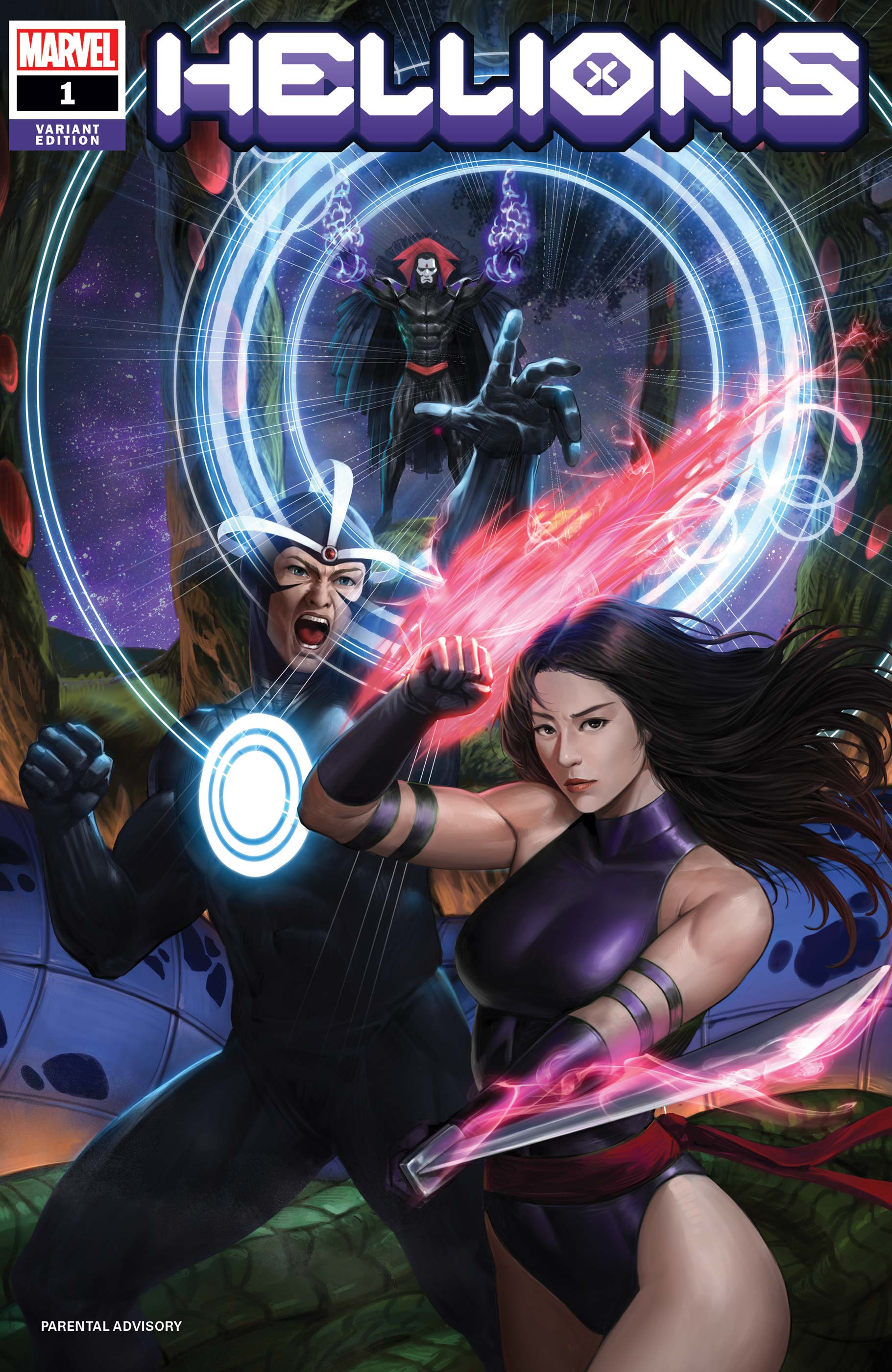The image depicts a vividly detailed comic book cover titled "Hellions Marvel 1 Variant Edition." Dominating the scene are three superhero characters, with the woman positioned prominently in the front right corner. She sports a striking purple leotard and black gloves, with vibrant pink energy emanating from her fists. To her left in the background, a man is seen, his helmet illuminated with a white glow and a white shield emblazoned on his chest. Additionally, another figure stands in the back right, emitting electric-like energy from their arms. The overall color scheme of the cover blends shades of purple, blue, black, off-white, and red, set against a backdrop of a purple sky. The white and purple text of the title "Hellions" is prominently displayed, and the cover bears the Marvel logo and a parental advisory warning in the left-hand corner, indicating this is indeed a Marvel superhero comic book. Subtle details such as the wristbands on the woman's arms and the glowing circle on another character's chest further enhance the dynamic and heroic essence of the illustration.